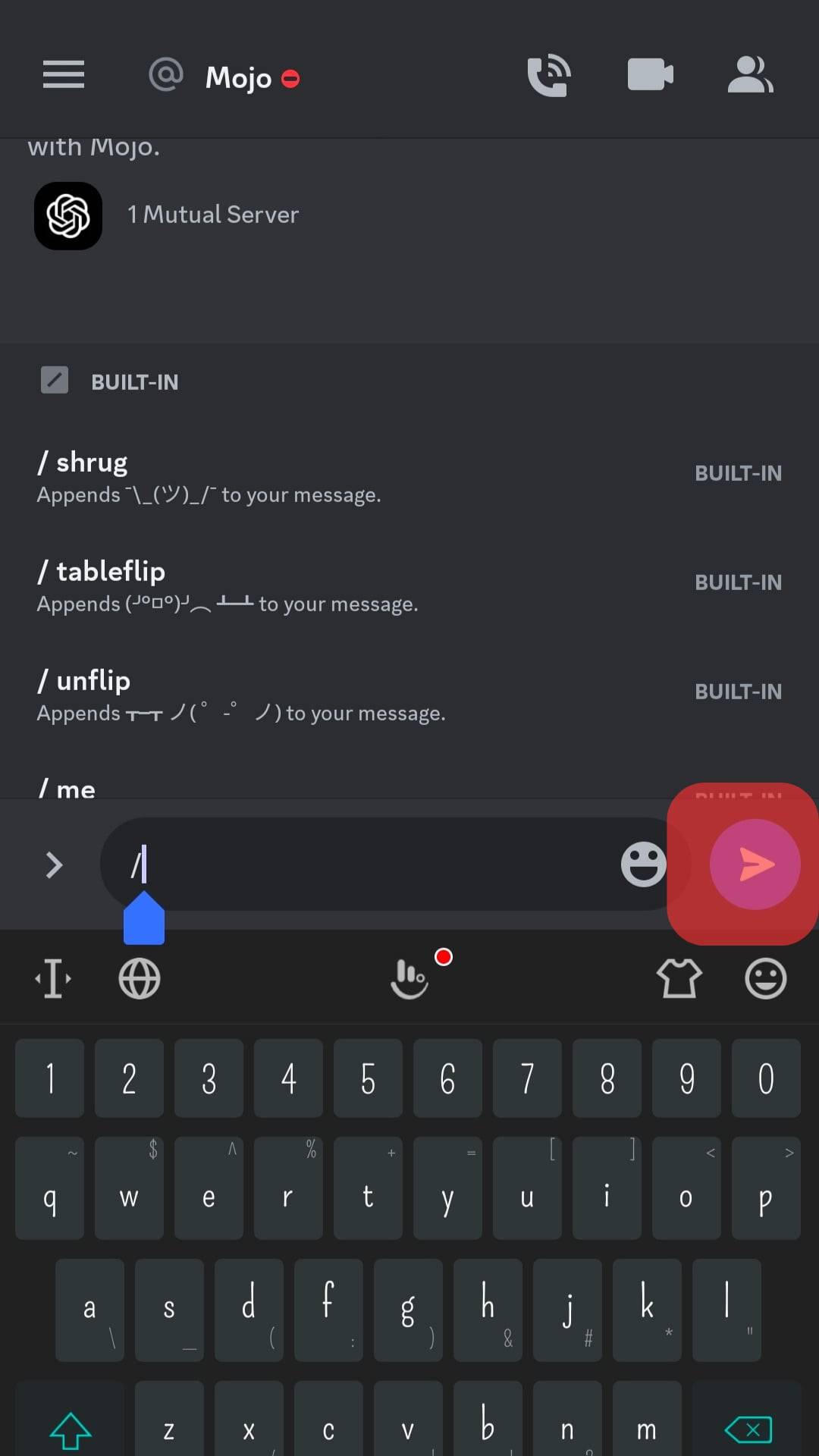The image features a mobile phone screenshot displaying a dark-themed interface, likely from a messaging or social app. The background gradient transitions from black to light gray. At the top of the screen, the title "Mojo" is prominently displayed, indicating the app's name, accompanied by the phrase "with Mojo." A small icon beside the title denotes "one mutual server," suggesting a server-based communication platform. 

In the top navigation bar, typical mobile icons such as three horizontal lines (menu), a phone, a camera, and a profile icon are visible, confirming it's a mobile viewpoint.

Below this, the screen lists various emoticon shortcuts and their descriptions:
- "built-in" followed by "#shrug" and the text "appends the shrug icon to your message."
- "table flip" followed by the text "appends the flipping table icon to your message."
- "unflip" followed by "appends the unflipping table icon to your message."
- "/me" followed by a search bar where users can type and search for specific commands or emojis.

The display also shows an active keyboard in dark mode, featuring a light black background with dim, turquoise-tinted keys. This color scheme gives the interface a sleek, modern look. The image overall focuses on the in-app interface and functionalities available for user interactions.